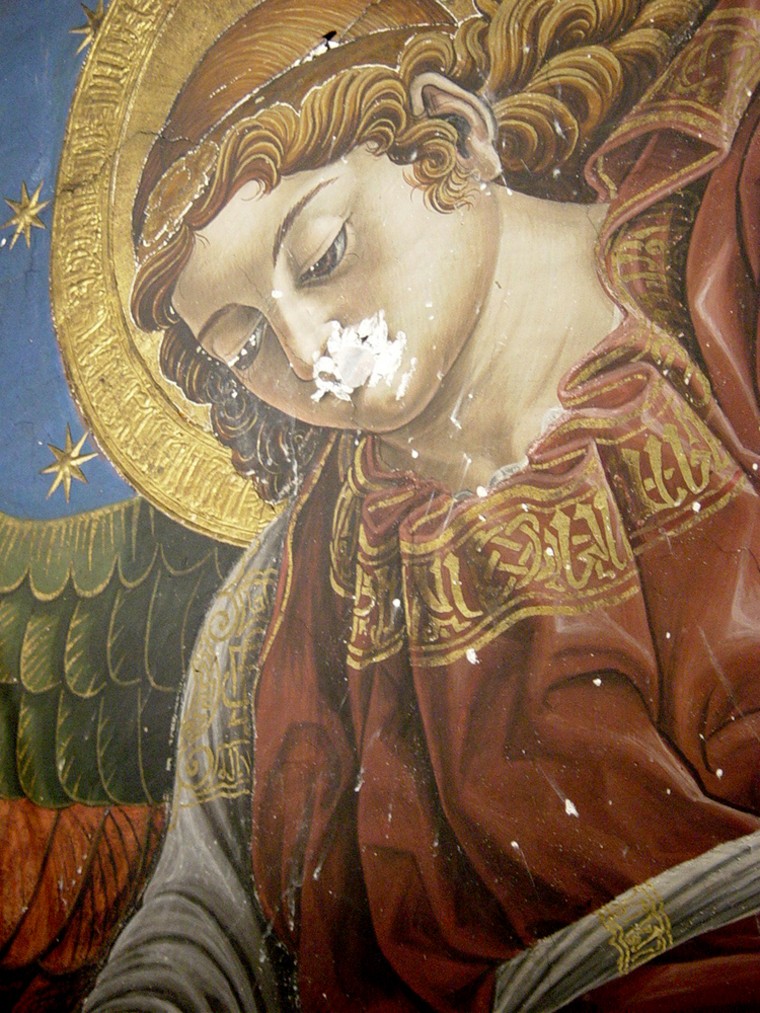In this painting, which appears to be from the early Renaissance period, a woman, possibly an angel, is depicted in a damaged fresco. The artwork shows signs of age, with cracks and chipped paint revealing deterioration. The woman is seated and shown from head to waist, adorned in a red gown with gold decorations around the neckline. A white belt cinches her waist, and her long, curly blonde hair cascades in ringlets almost to her shoulders. A gold halo encircles her head, suggesting a divine or saintly figure. Notably, a single wing extends from her left side. The background features a blue section with golden stars and a gold emblem, along with green flaps reminiscent of turtle scales.